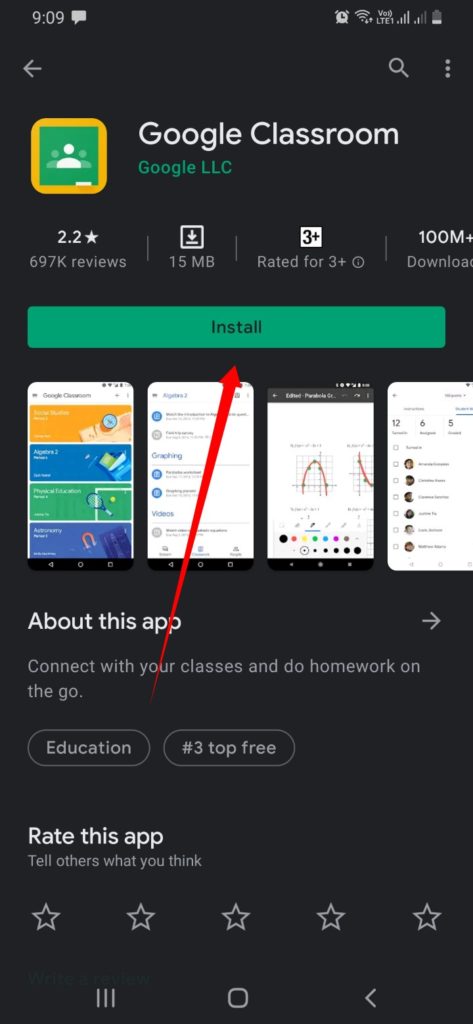This image is a screenshot from a phone displaying the Google Classroom app on the Google Play Store. At the top, the screen shows "Google Classroom" with "Google LLC" written below it in green text. Adjacent to this is a green square icon bordered with a yellow-gold line.

Below the app's name, the rating is displayed as 2.2 stars, followed by a detail indicating the app size of 15 MB. It mentions the app is rated for ages 3 and up and highlights that it has over 100 million downloads. The green "Install" button, with the word "Install" in black text, is prominently featured.

The background of the screen is black, showcasing three or four promotional images demonstrating various uses of Google Classroom. An arrow extends from the phrase "about this app," moving through the word "your" in the phrase "connect with your classes and do homework on the go," and pointing towards the "Install" button.

At the bottom of the screenshot, it notes that the app falls under the "Education" category and is tagged as "#3 Top Free." There is also an option to rate the app with stars.